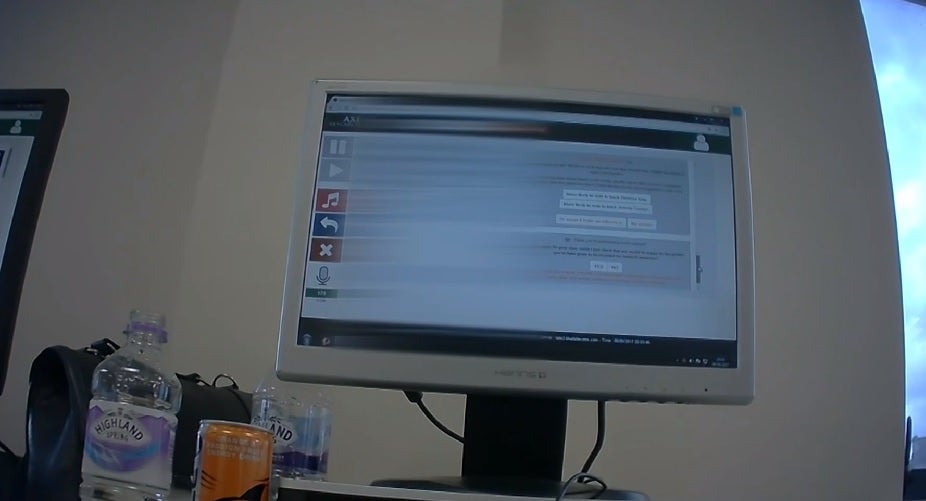In the image, an off-white wall serves as the backdrop. Positioned centrally is a grey monitor featuring a black screen that is currently off. To the bottom left of the scene, several plastic Highland bottles are visible, distinguishable by their purple and blue accents with partially visible black lettering spelling "Highland."

In front of these bottles, an orange can with white lettering stands prominently. Another black screen is partially visible to the left, discernible by a black line, white circular icon at the top, and shoulder icons underneath.

The grey monitor's screen displays a black banner on the right, featuring a white head and shoulders icon. To the left, set against a white and grey background, are various control icons including a pause button, play button, a music note icon, a back arrow icon with a blue background, an X icon with a red background, and a microphone icon.